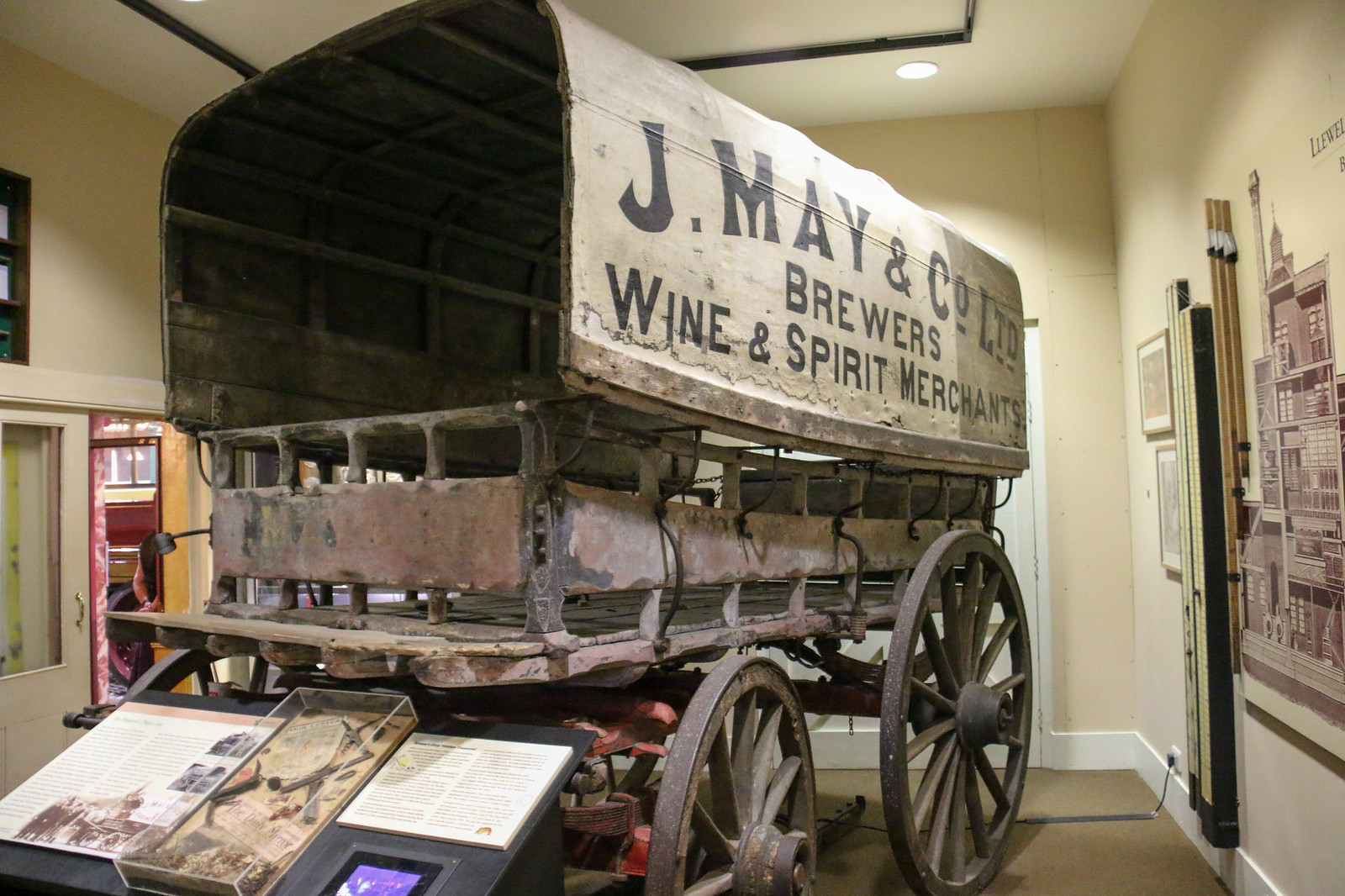The image depicts a large, old wagon, likely from the early 1900s, prominently displayed in the center of a carpeted room which seems to be part of a museum exhibit. The walls of the room are beige, and a door on the left allows natural light to flow in. The wagon, which bears the moniker "J. May and Company Brewers, Wine, and Spirit Merchants" on its side, is covered in a white canvas with blackish lettering. The vehicle has large, old spoke wheels and appears to be quite aged and rusty. Surrounding the wagon, there are several pictures and artworks hanging on the walls, including a picture of a city visible on the right side of the image. In front of the wagon, there is a see-through display box likely explaining the history of J. May & Co., along with some related tools. Light fixtures on the ceiling illuminate the exhibit, highlighting the intricate details of this historical vehicle.